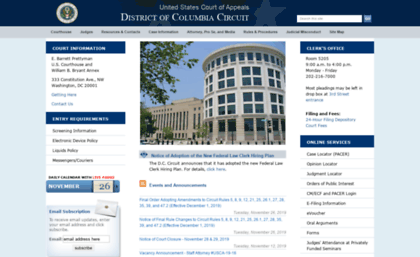The image is a small, horizontally rectangular screenshot of the United States Court of Appeals for the District of Columbia Circuit. At the very top, a dark blue horizontal banner features the court's name in white text, centered prominently. The official seal of the court is visible on the left side of the banner, though the small size of the image renders it indistinct. 

Below the banner, the focal point is a photograph of the courthouse building, positioned centrally. Flanking the courthouse image are two columns of text under headings that are also on blue banners, with their individual items listed underneath on a white background, though details are not discernible due to the image size. Directly beneath the courthouse picture, a series of additional links are displayed in blue text, but they are too small to read clearly.